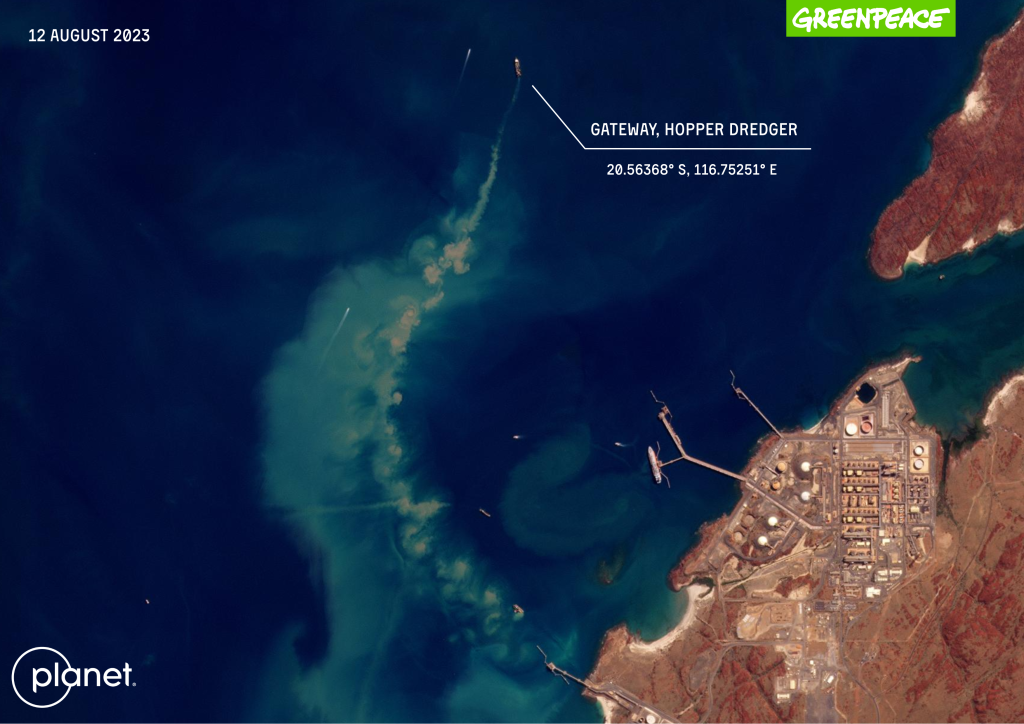An aerial view of a coastal area is depicted in this detailed map image. The map is highly zoomed out, showcasing a predominantly brown landmass on the right side, indicating a settlement area with visible rooftops, roads, and buildings. This land is bordered by a deep blue sea, exhibiting a gradient of blue shades, from dark to light. Near the bottom right, there is what looks like a docking area with several small boats and a prominent ship labeled "Gateway Hopper Dredger," highlighted with white directional lines pointing to its exact coordinates: 20.56368 degrees south, 116.75251 degrees east.

Inscriptions mark various places on the map: The date "12 August 2023" appears at the top left in white font. The top right bears the label "Green Peace" in white lettering set against a light green background, and just beneath it, the coordinates and name of the highlighted ship are displayed. Finally, the bottom left features a planet icon with a stylized text, where the letters "P" and "L" are encircled starting from the letter "A."